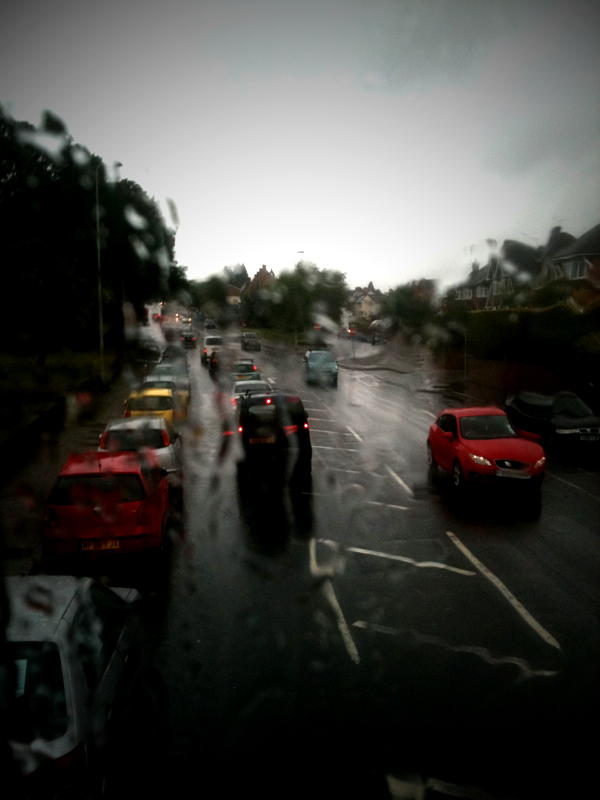The image depicts a one-lane road stretching towards the camera under a gray, stormy sky, indicative of a recent rainfall. The pavement glistens with wetness, though it is not currently raining, suggesting the photo was taken shortly after a downpour. A long line of cars is parked on the left side of the road, adjacent to a tan-colored sidewalk and a row of green trees. Amid this, a black car is prominently visible. On the right side of the road, traffic moves towards the camera, with a red car leading and followed by a blurry blue car. In the distance, the right side of the scene features houses and additional trees, all slightly out of focus. White line markings on the blacktop enhance the visibility of the road. The overall ambiance of the image is dominated by the stormy, wet conditions and the contrasting colors of the cars, which range from black and white to red, yellow, and blue.